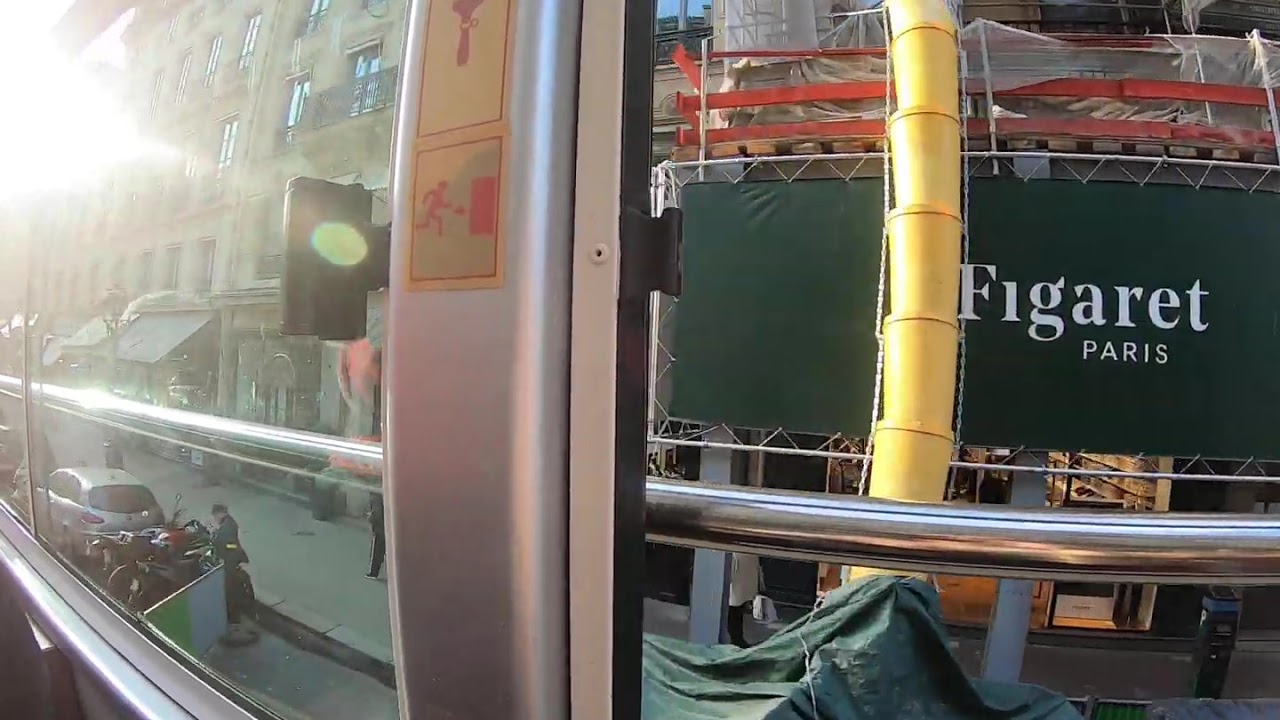The image depicts an elevated vantage point, possibly from a bus or train window, looking out onto a Parisian street. Prominently featured is a dark green sign with white lettering that reads "Figarette Paris." Close examination of the scene through the large glass panes, divided by a silver beam with a potential emergency exit symbol, reveals a bustling sidewalk below. The sidewalk is populated with parked motorcycles, a van, and a couple of cars. A beige building lines the street, adorned with awnings of various businesses. There is visible construction, evident from a tarp covering part of the storefront and plastic tape running above the sign. Among the pedestrians, one person is seen holding a white bag, and another stands near a motorcycle. The scene captures the essence of an urban Paris landscape with its mix of commerce and everyday street activity.